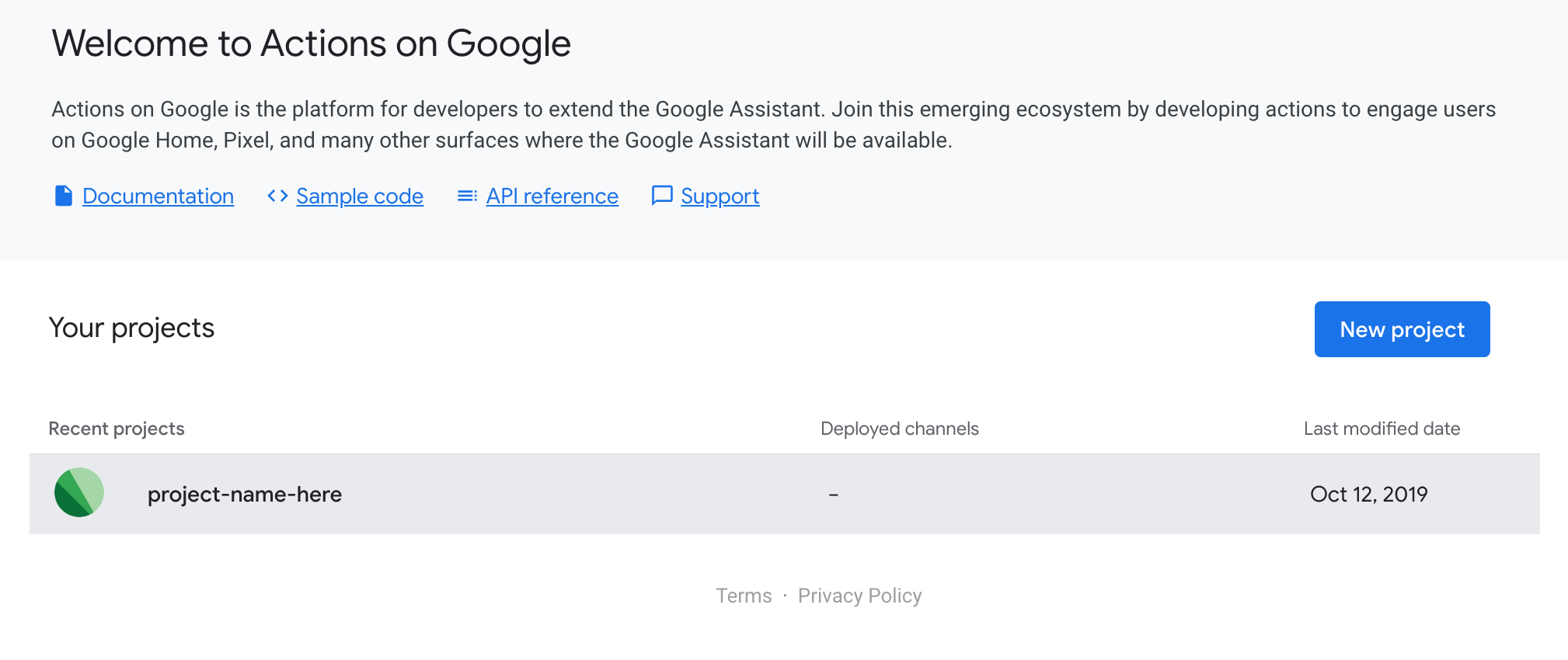The image is a webpage from Google, specifically showcasing "Actions on Google," a platform for developers to extend functionalities of the Google Assistant. The background transitions from a light gray at the top to white.

At the top left, in bold black text, it states, "Welcome to Actions on Google." Below this, a brief introduction explains that Actions on Google is a platform for developers to create actions to engage users on Google Home, Pixel, and other devices compatible with Google Assistant.

Under this introduction, there are four blue hyperlinks, each accompanied by an icon:
1. "Documentation" with a document page icon.
2. "Sample Code" with left and right brackets icon.
3. "API Reference" with a hamburger menu icon.
4. "Support" with a chat box icon.

Further down, a heading in black text reads, "Your Projects," with a blue button to the right labeled "New Project" in white lettering. Below this are sections titled "Recent Projects," "Deployed Channels," and "Last Modified Date."

In the "Recent Projects" section, there is a gray box featuring a blue circle with varying shades of green on the left, labeled "Project Name Here." The "Deployed Channels" section shows a dash, and the "Last Modified Date" reads "October 12, 2019." At the bottom of the page, the terms "Terms" and "Privacy Policy" appear in gray text.